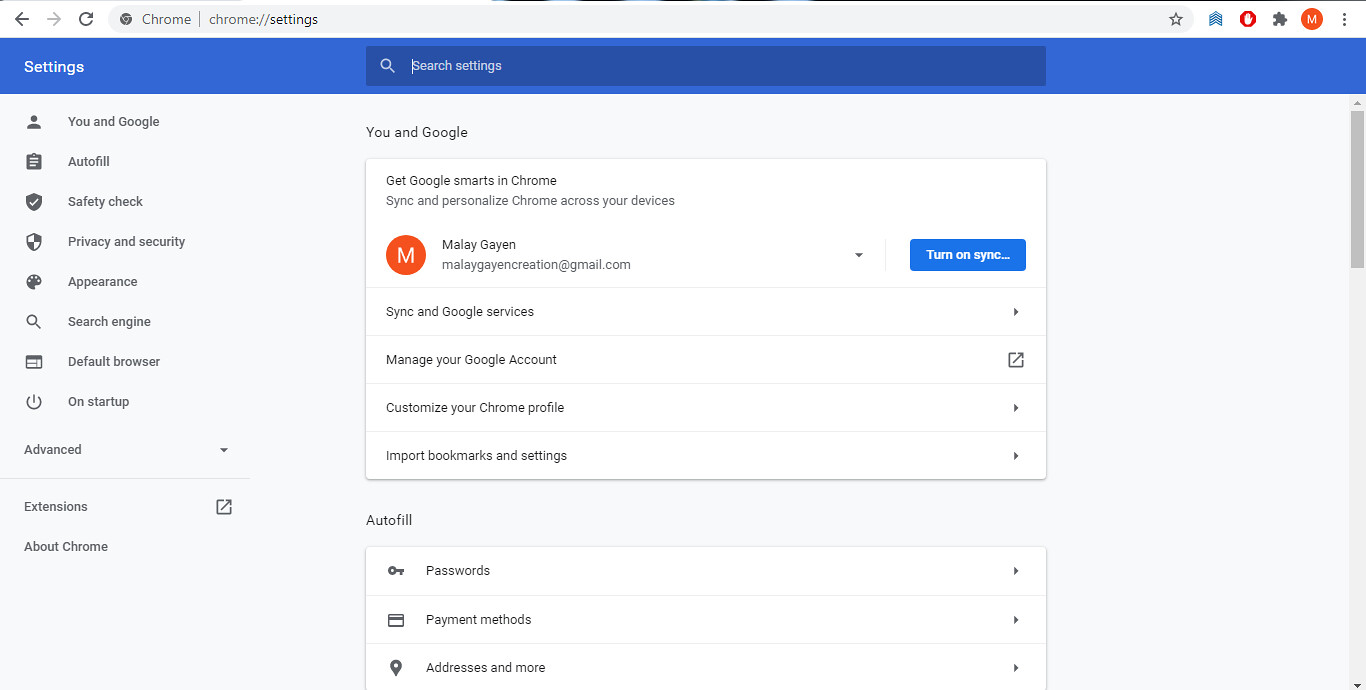This image captures a Google Chrome settings page, specifically displaying options to manage and customize a Google account within the browser. Dominating the upper portion, a search bar is visible, aiding in quick navigation through the settings. Just beneath it, various Chrome settings categories are listed: "Autofill," "Safety," "Privacy," "Appearance," "Search Engine," "Default Browser," and "Startup," along with an expandable "Advanced" section denoted by a downward arrow. Options for "Extensions" and "About Chrome" are also shown.

The central focus is on the "Turn on Sync" feature, with text encouraging users to leverage Google's synchronization capabilities to enhance their browser experience. Displayed prominently are the name and email of the individual logged in: Melee Gayen (melee.creation@gmail.com). Underneath, there are controls for "Sync and Google Services," "Manage your account," "Customize your Google profile," and options to import bookmarks, along with settings for passwords, payments, and addresses.

In the upper corner of the interface, a red-circled "M" icon represents the user's profile, alongside a star icon. To the far upper right, there are three vertical dots forming a menu for additional account management options, as well as a small dark cloud icon indicating the presence of additional Google applications.

The page features a clean white background with red and blue highlights, reflecting Google's minimalistic design ethos for a user-friendly interface.